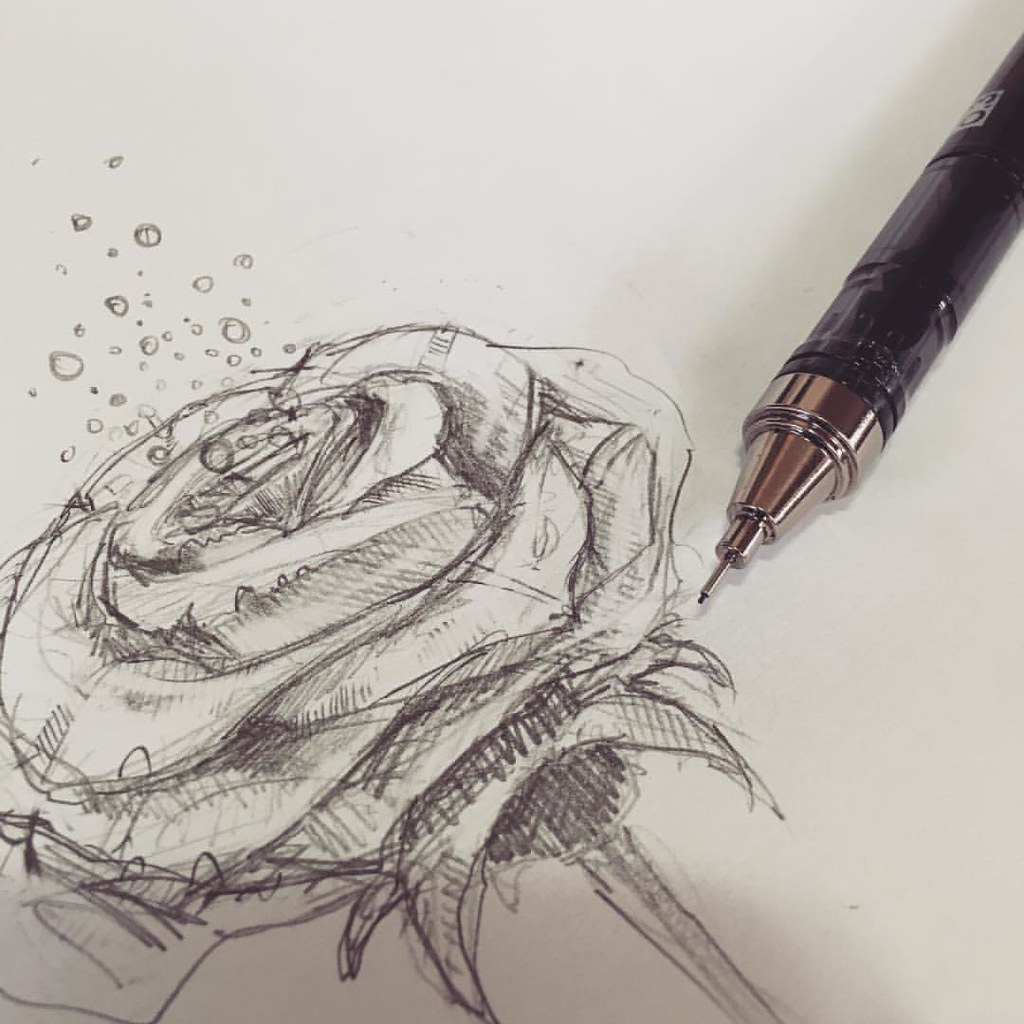A meticulously detailed pencil drawing of a rose is captured within this square image, set against a pristine white background that mimics the appearance of clean white paper. The drawing is executed with a mechanical pencil featuring a sleek black body and a silver tip, from which a small segment of black lead protrudes. This pencil is positioned diagonally in the upper right corner, pointing towards the center, encroaching into the visual space of the rose artwork. The rose itself is exquisitely rendered with intricate details, depicting delicate petals and subtle water droplets that appear to emerge from its core. The drawing includes a partial view of the stem, extending halfway down, contributing to the overall realism and intricacy of the illustration.